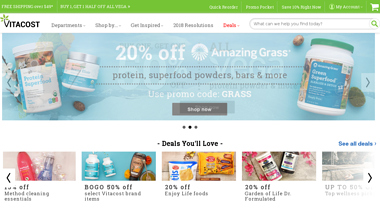Here is a detailed and cleaned-up caption for the image:

"The image showcases the upper section of the VitaCost website, adorned with a vibrant green banner stretching across the top. This banner highlights special promotions and offers, such as 'Free Shipping Over $49' and 'Buy One, Get One, Half Off All FICA.' Key navigation links like 'My Account' and a 'Save 20%' notification are also present. Below the green banner, there is a secondary teal background featuring promotions for protein superfoods and organic superfoods, including an offer of '20% Off Amazing Grass.' This section specifically advertises protein superfood powders, bars, and more, encouraging customers to 'Use Promo Code GRASS' (G, R, A, S, S in capital letters). Below this, a prominent gray 'Shop Now' button invites users to explore further. The 'Deals You'll Love' section offers various discounts such as 'Buy One, Get One 50% Off,' additional '20% Off' offers, and a specific '20% Off Garden of Life' promotion."